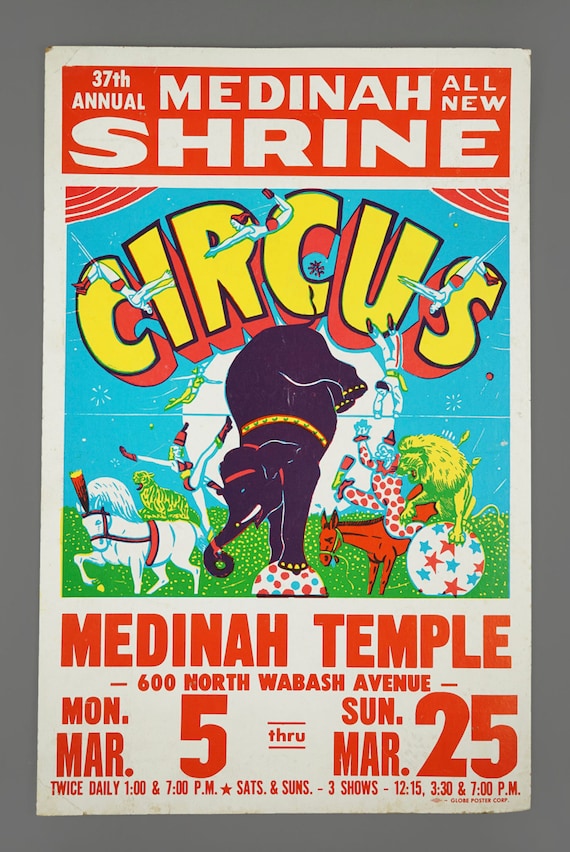The image depicts a color photograph of a rectangular circus poster set against a dark grey border. The upper portion of the poster features a red header with white text that reads "37th Annual Medina All New Shrine." Below this header, prominently displayed in an arching manner, is the word "CIRCUS" in bold, 3D yellow letters outlined in black. The background behind "CIRCUS" is blue, further highlighting the text.

The main visual content of the poster includes a vibrant depiction of various circus acts: a black elephant balancing on a ball with its front legs while another performer stands on its trunk, a green lion perched on another ball, and several horses, including a brown horse ridden by a clown and a white horse performing stunts. Additionally, there are acrobats and trapeze artists engaged in mid-air feats above the animal performers, all set against a green backdrop that suggests an outdoor setting with grass.

The lower third of the poster provides details about the event, listing "Medina Temple, 600 North Wabash Avenue" as the venue. The event runs from Monday, March 5th through Sunday, March 25th, featuring showtimes set at 1 PM and 7 PM daily, with additional shows on Saturdays and Sundays at 12 PM, 3:30 PM, and 7 PM.